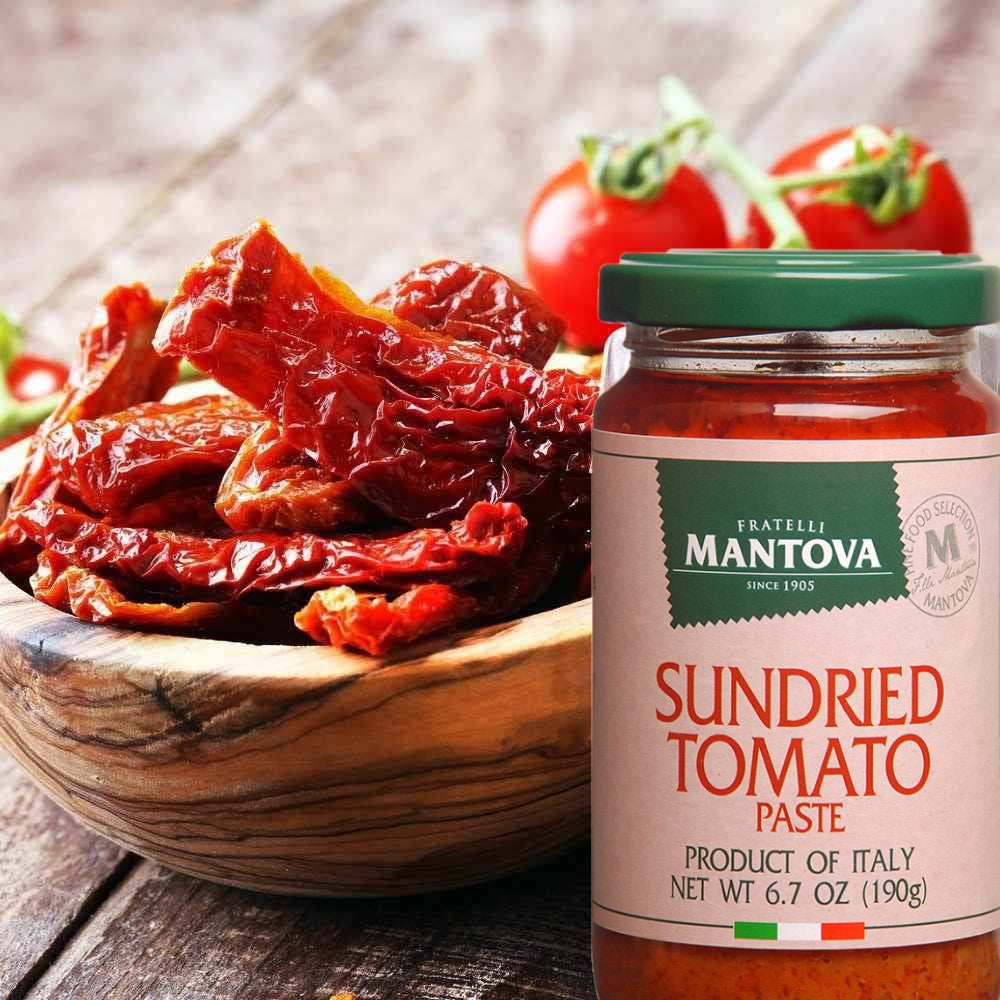This vibrant color photograph showcases a meticulously arranged culinary scene set on a rustic, distressed wooden surface in a grayish hue. Dominating the foreground toward the right, a clear glass jar of Fratelli Mantova sun-dried tomato paste takes center stage. The cylindrical jar, capped with a green metal lid, features a white label adorned with intricate details. At the top of the label, against a green background, the text "Fratelli Mantova since 1905" is prominently displayed in white lettering. Below this, "sun-dried tomato paste" is vividly written in red on the beige section of the label, followed by "product of Italy" in green, and the net weight "6.7 oz (190 grams)" in black. A small tricolor band in green, white, and red reminiscent of the Italian flag adorns the bottom of the label, reaffirming its authentic Italian heritage.

To the left of the jar, enhancing the composition, is a rustic wooden bowl brimming with sun-dried tomatoes. These tomatoes, with their shriveled, bacon-like appearance, vary in shape, some being long and thin while others are chunkier. Providing a vibrant contrast, a vine of fresh whole red tomatoes lies in the background, slightly out of focus, further enriching the composition. The entire scene is an evocative visual narrative that highlights the rich textures and colors of Italian cuisine ingredients.